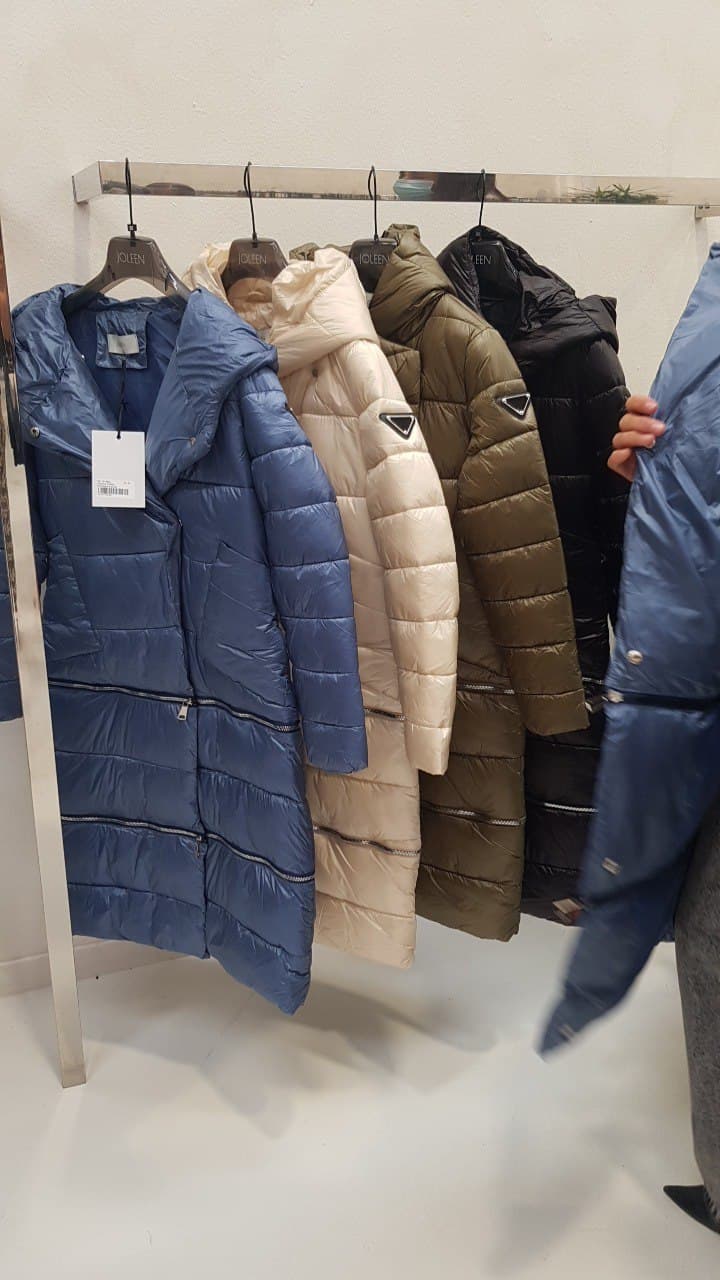The photograph captures a wall-mounted, silver metal rack situated in a store with an all-white floor. The rack displays four full-length, puffy winter coats, known as "marshmallow coats," hanging from sturdy hangers. The coats, which come in diverse colors—blue, white, bronzy brown, and black—are identical except for their hues, all featuring a black, upside-down triangle logo on the left sleeve, signifying the same brand. The blue coat on the far left still has a white tag attached, although the text is not legible due to distance. To the right of the rack, partially in view, stands a woman wearing a blue mask, in the process of donning a blue puffy coat, visible in the rack's reflection. Each coat includes a zippered section that allows them to be adjusted for length, emphasizing their functional design.